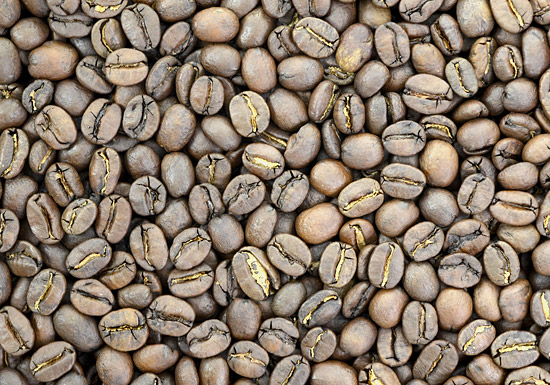This landscape-oriented photo features a densely packed layer of dried, unroasted coffee beans covering the entire frame. The beans exhibit a range of shades between tan, gray, and light brown, giving them a raw, frosty appearance. Some beans are whole and intact, while others are slightly cracked, revealing a yellowish interior. These creases, visible on about half of the beans, hint at a golden hue when illuminated. The uniformity in their color varies slightly, with a subtle mix of darker and lighter tones among the beans. The overall well-lit scene highlights the intricate textures and details of the beans, presenting them freshly harvested in a natural, untouched state.